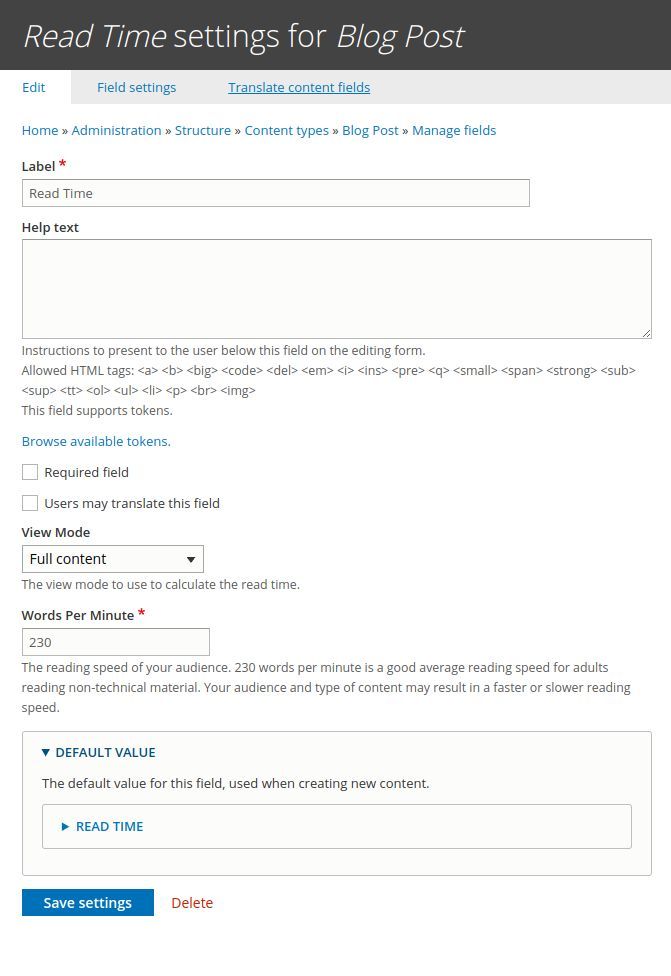The image displays a webpage titled "Read Time Settings for Blog Post," prominently positioned at the top. Beneath the title are three blue-colored links: "Edit," "Field Settings," and "Translate Content Fields." The page contains several sections where various types of information can be entered. Key labels include "Label," "Help Text," "View Mode," and "Words Per Minute," suggesting a settings page for blog post configurations on a website.

The page's background is solid white, and most of the text is black, except for the blue links. At the very bottom left corner, there are two buttons: a blue "Save Settings" button and a "Delete" button located to its right. The array of editable fields and options throughout the page indicates comprehensive customization capabilities for blog post settings.